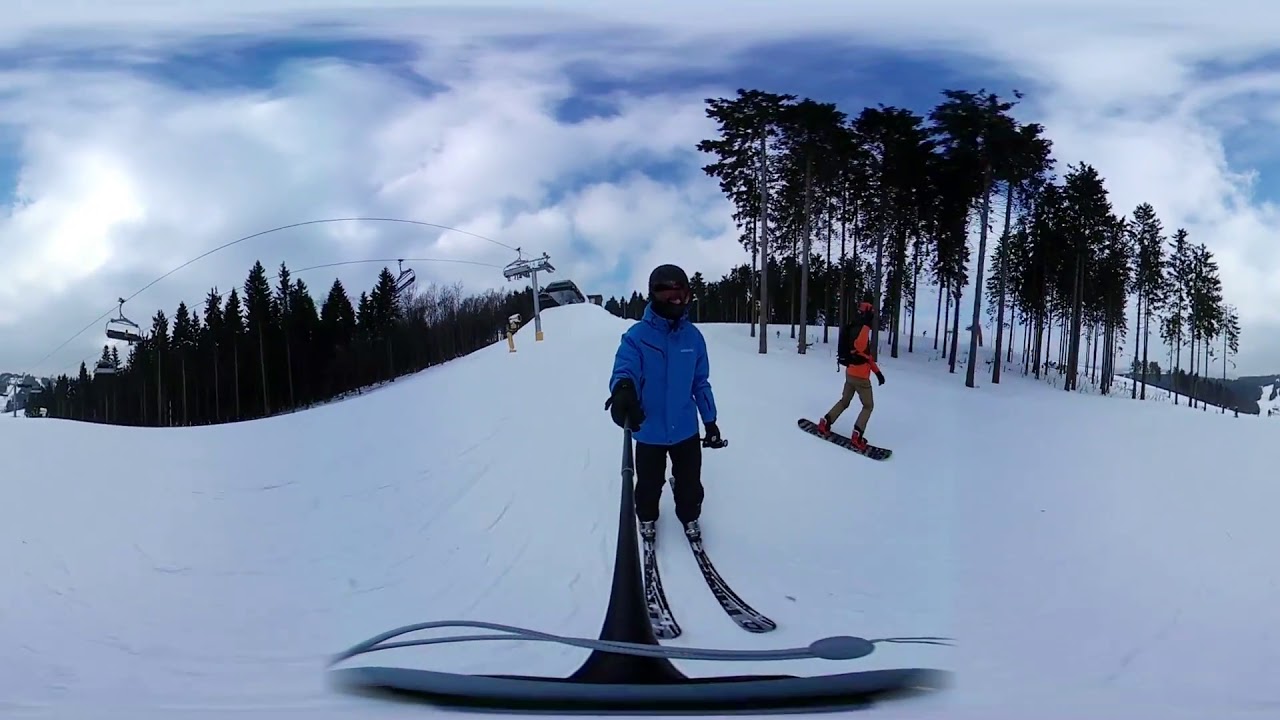In this vibrant image captured from a skier's selfie stick, two outdoor enthusiasts are seen descending a snow-covered mountain slope. The person in the forefront, sporting a blue jacket, black pants, black skis, and a full-faced helmet with a black scarf or mask, is capturing the moment as he skis downhill. He is holding the selfie stick with black snow gloves, providing a dynamic perspective of the scene. Beside him, his partner snowboards down the hill, clad in an orange and black jacket, tan pants, and a blue backpack. His black snowboard, marked with red writing, contrasts with the snow. The backdrop reveals a sprawling ski slope stretching into the distance, flanked by a mix of tall, dark evergreen trees and other towering, sparse trees. A ski lift, devoid of passengers, hovers in the background against a predominantly cloudy sky with hints of blue peeking through. The shot encapsulates a lively scene full of colors, including black, white, green, grey, blue, orange, and brown, embodying the thrill of skiing and snowboarding amidst nature.